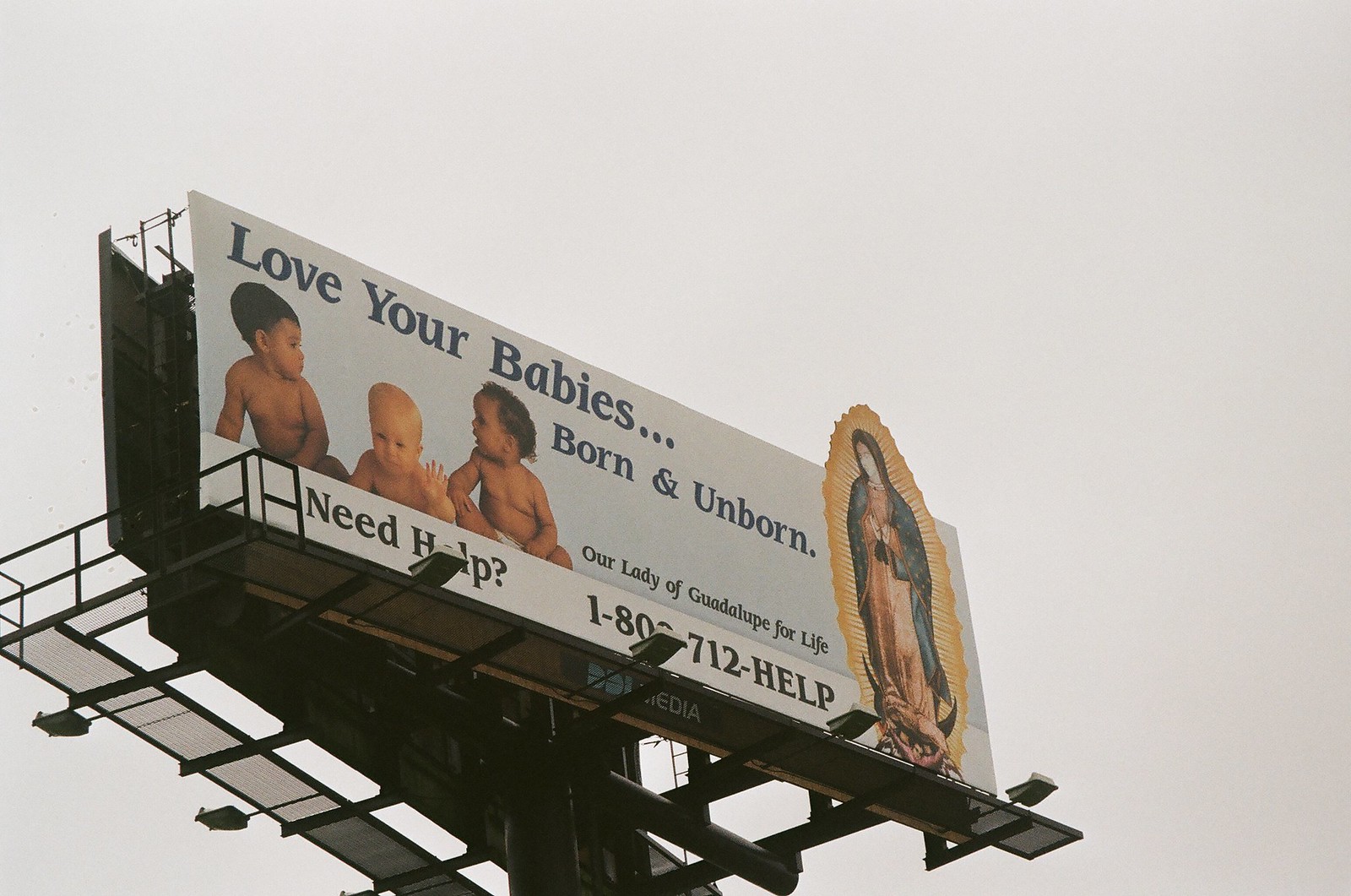This outdoor photograph captures a large metal-framed billboard set against a gray, overcast sky. The billboard, supported by a substantial black structure, features a catwalk, a ladder, and lights along its bottom edge, indicating it can be illuminated at night. The center of the billboard displays an image of three babies: a white baby with ginger hair waving at the camera, an Asian-looking baby on the left, and a black baby on the right. Above them, large text reads, "Love your babies, born and unborn. Our Lady of Guadalupe for life." To the right of the babies’ image is a picture of the Virgin Mary with an orange halo. The bottom portion of the billboard has a white stripe with black text, stating, "Need help? 1-800-712-HELP." This advertisement appears to be promoting a pro-life message, as inferred from the imagery and text.